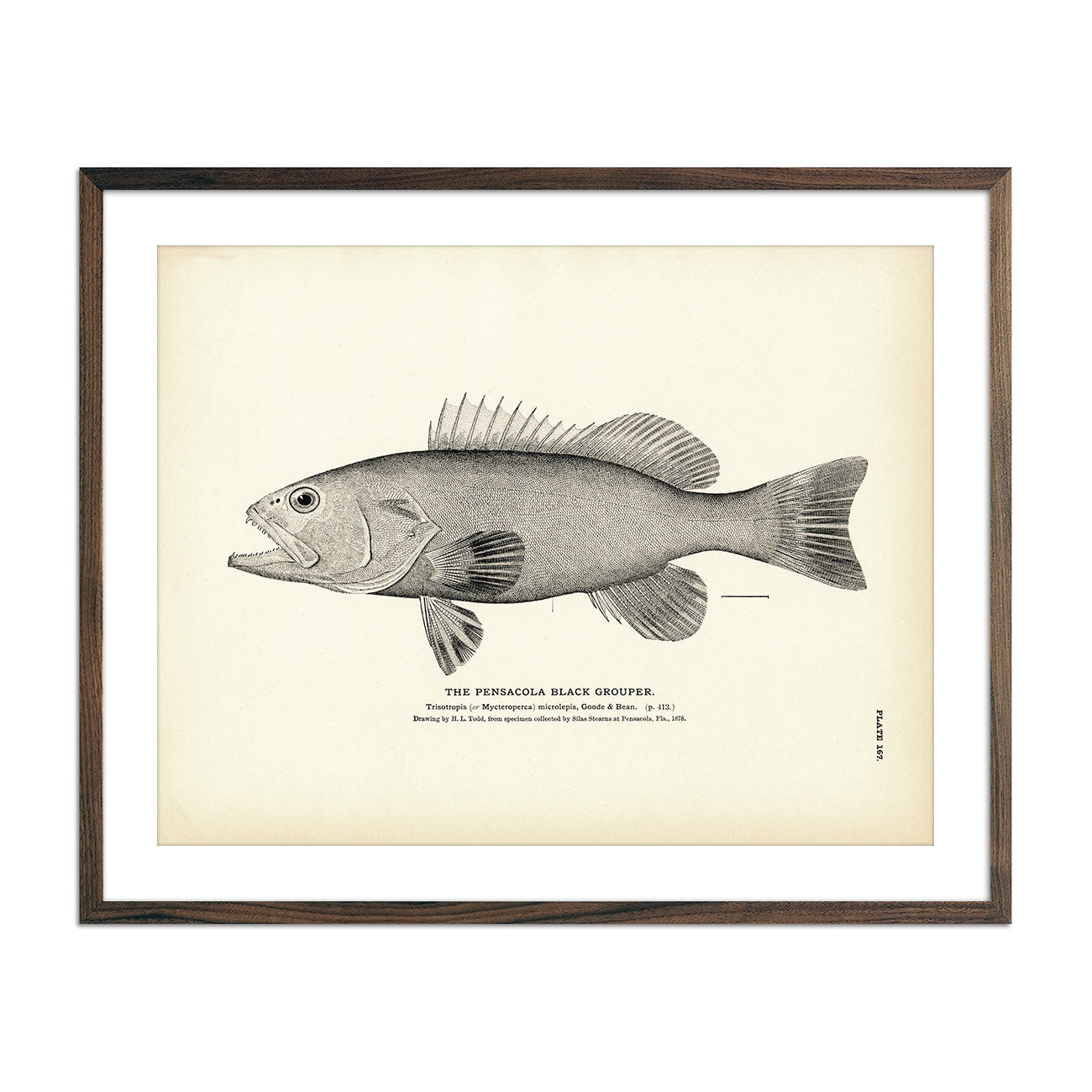Framed elegantly in a darker, faded brown wood, this large poster showcases a remarkably detailed pen drawing of a fish, prominently displayed against a pristine white background. The fish sketch is meticulously executed in black ink on cream-colored paper, capturing lifelike nuances through very fine pen strokes. Surrounding the illustration is a clean white border that adds a touch of sophistication.

The fish, identified as the "Pensacola Black Grouper," is rendered with exquisite accuracy, from its multiple pectoral fins to its spiny dorsal ridge. Its mouth is open, revealing pointed needle-like teeth, enhancing the realism of the drawing. Beneath the fish, there is descriptive text, including its Latin name and a reference to the plate number "167," suggesting that this artwork is an excerpt from a textbook. Although the artist's name and possible location are partially obscured, the skill and detail evident in the drawing underscore the artist's dedication to capturing the essence of this marine creature.